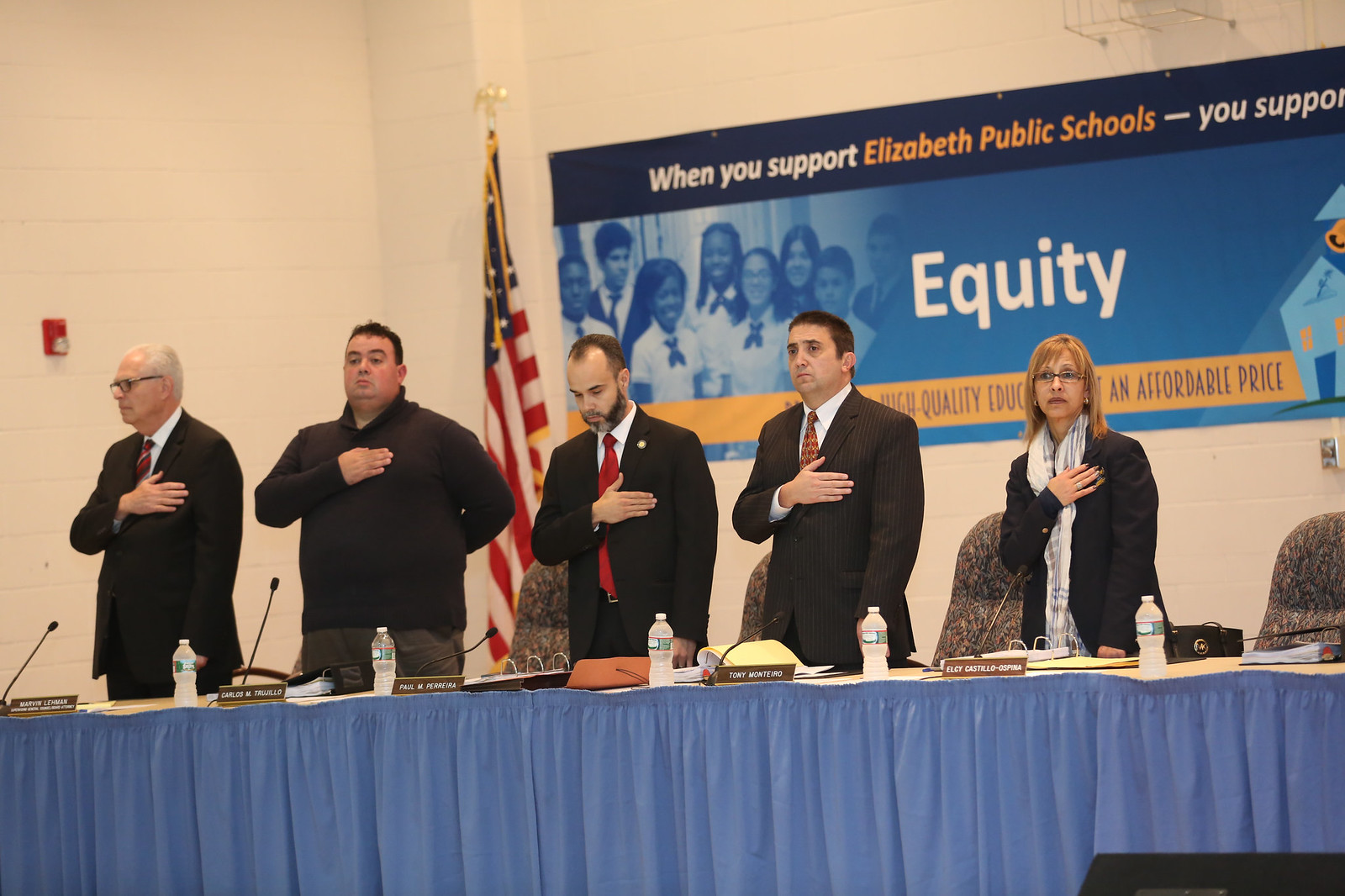The image shows five people standing behind a long banquet table draped with a blue cloth. They are all dressed in business attire, with the most casual outfit being a black zip-up jacket. On the left, an older gentleman with graying hair is wearing a black coat jacket. Next to him stands a heavier set man in his 30s, dressed in a black zip-up jacket. The third person is a slightly balding man with a graying beard, wearing a black suit jacket and a red tie. The fourth person appears to be in his 40s and wears a black suit jacket with vertical stripes and a decorated red tie. The woman on the far right is short, wearing a black suit jacket with a scarf.

In front of each person are nameplates and microphones, suggesting a formal setting, likely a committee convening. They are standing with their hands over their hearts, as if for the Pledge of Allegiance or the National Anthem. Behind them is an American flag on the left and a sign reading, "When you support Elizabeth Public Schools, you support equity," with the word "equity" prominently displayed in large white letters.

From left to right, the nameplates identify the individuals as Marvin Lindman, Carlos M. Trujillo, Paul M. Perroa, Tony Montero, and Elsie Castillo Ospina.